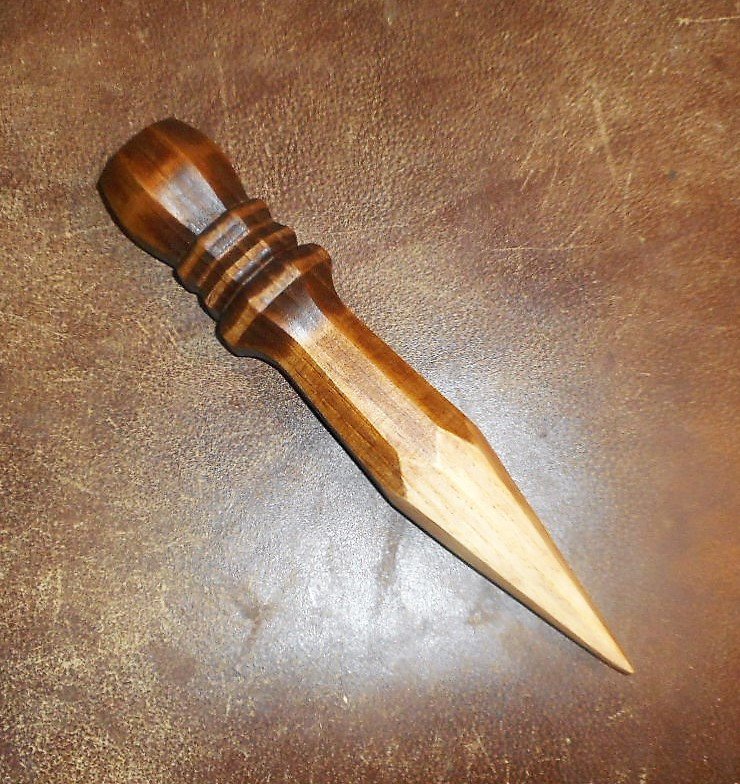The image features a highly polished wooden stake, meticulously crafted from different shades of wood. The stake transitions from darker wood at the base, through medium tones, and tapering to a very light, sharply-pointed tip. The stake is positioned diagonally, with the tip pointing to the bottom right of the picture and the head oriented towards the top left. The smooth, carefully carved handle displays a series of jagged, yet polished designs below it, adding to its elaborate craftsmanship. The background is a brownish, leather-like material adorned with subtle markings and hints of burgundy and beige, providing a contrasting texture to the wooden stake. The object resembles a leg of a chair or a carved post, possibly even reminiscent of a bed frame pole, further emphasizing its multifunctional potential and elegant design.